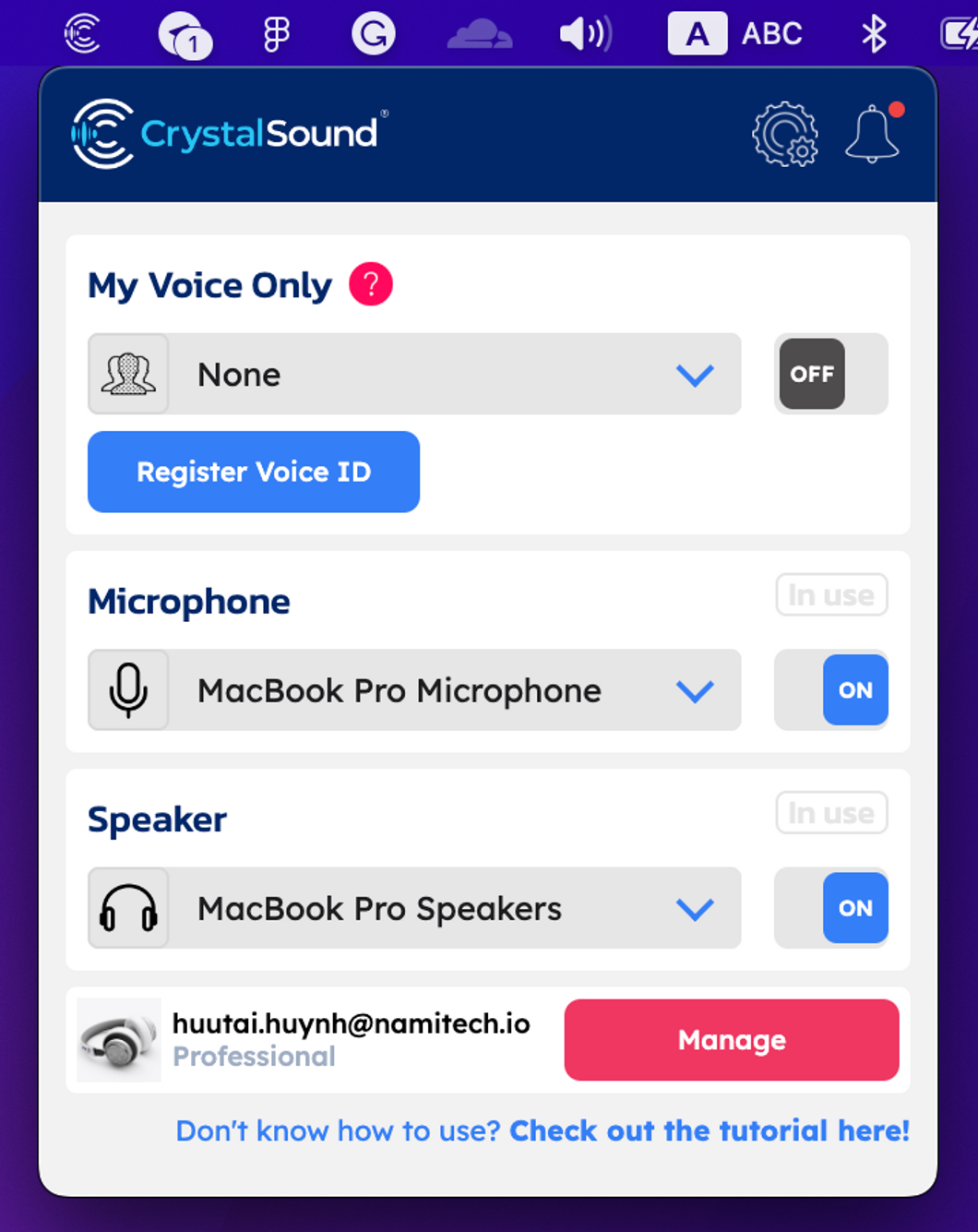The image appears to be a rectangular screenshot of an application interface. In the upper left corner, there's an app icon consisting of a series of white circles nested within each other, divided on the right side, set against a dark blue background. Adjacent to the icon, the brand name "Crystal" is written in light blue text followed by "sound" in white text.

At the top of the screenshot, several icons are visible, primarily white in color. A cloud icon with a gray hue appears roughly at the center, while to the right, a partially visible battery icon outlined in dark blue features a white lightning bolt in its center.

Below the header reading "Crystal sound," various options are presented. A dark blue text label reads "My voice only," positioned next to a red circular icon with a white question mark at its center. A gray rectangular drop-down menu labeled "None" is visible beneath this.

Further down, a blue rectangular button with white text reads "Register Voice ID." Additional options for "Microphone" and "Speaker," each accompanied by individual drop-down menus, are also visible. The open menu has a predominantly white background, contrasting with the broader screen backdrop which exhibits a gradient effect shifting between purple and blue hues.